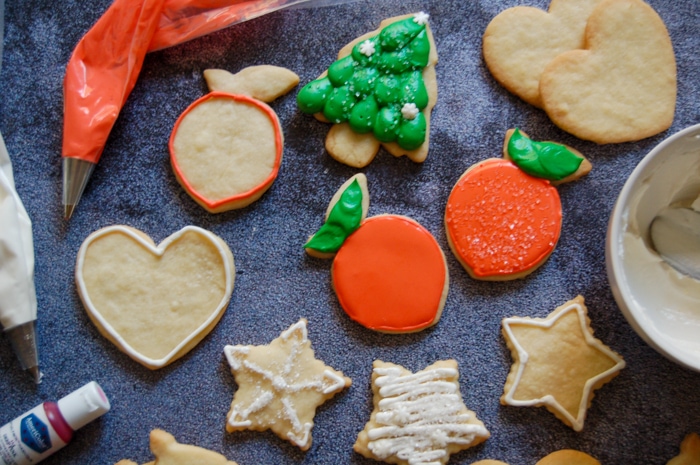The rectangular image, wider than it is tall, captures a delightful array of cutout cookies that appear meticulously arranged on a cloth-like blue surface. This setup bears a resemblance to vibrant holiday magazine spreads or social media baking posts. 

On the top right, the assortment begins with a pair of plain heart-shaped cookies beside a Christmas tree cookie adorned with green icing and white star decorations. Close by, two radish-shaped cookies showcase full orange coloring with green leaves, reflecting a playful take on classic cookie designs. Further left, another heart-shaped cookie is edged elegantly with white icing.

Below, three star-shaped cookies are artfully decorated with varied patterns of white icing. The scene includes practical baking elements as well, such as icing containers positioned on the left and food coloring in the bottom left corner, suggesting an ongoing decorating process. Intriguingly, a white bowl on the right holds white icing, paired with a spoon, ready for further cookie embellishment. This rich tableau, complete with its festive cookies and decorating tools, evokes a warm, creative vibe ideal for showcasing holiday baking adventures.